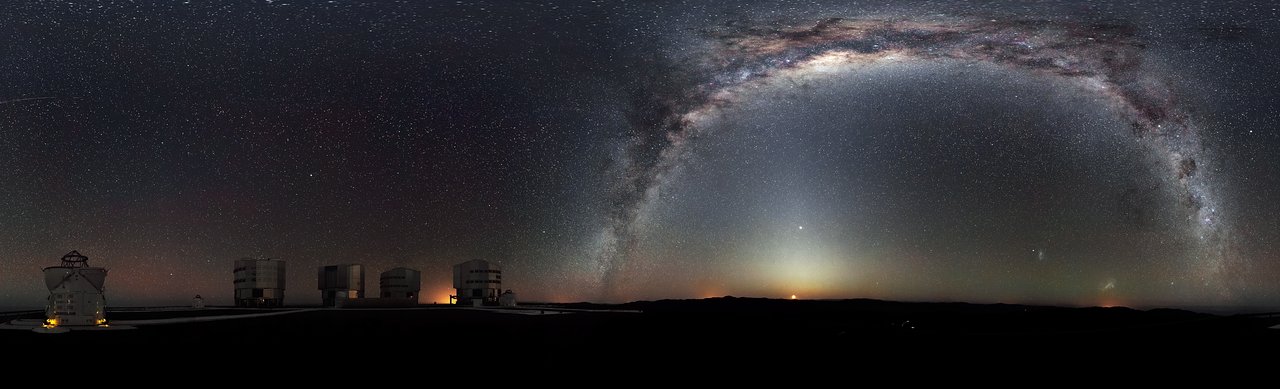This breathtaking wide-shot night skyline captures what appears to be the Milky Way galaxy, stretching across a dark sky filled with stars, free from any light pollution. The celestial display is awe-inspiring, with a half-circle of clouds partially illuminated, enhancing the scene's otherworldly beauty. Below, the ground is completely black, creating a striking contrast against the vibrant, star-filled sky. In the foreground, there are four cylindrical buildings with numerous windows, resembling futuristic towers, while a fifth, dimly lit building sits off to the left. The lack of contextual clues leaves the location a mystery, adding an enigmatic charm to this mesmerizing, potentially extraterrestrial landscape.